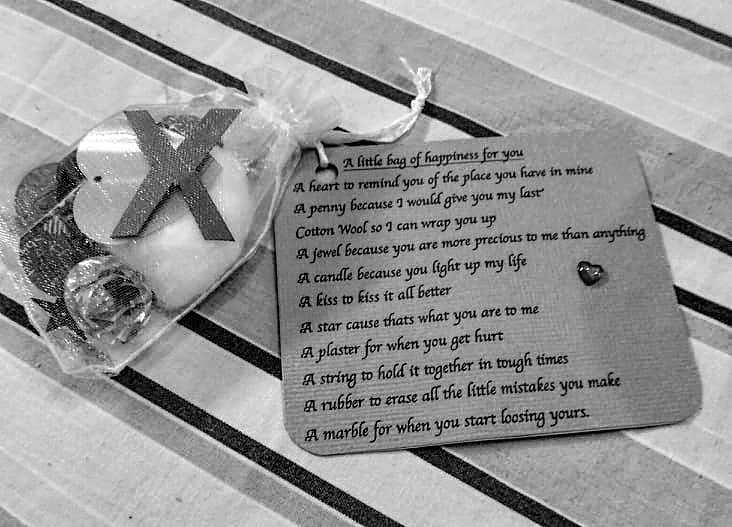This black and white photograph depicts a delicate party favor consisting of a small, see-through, mesh drawstring bag brimming with various items. Inside the bag, easily noticeable are a shiny heart and a letter X, among other indistinguishable goodies, potentially including a ball and other wrapped items. The bag is tied at the top with a string that also secures a rounded square tag with a heartfelt poem. The inscription reads: "A little bag of happiness for you, a heart to remind you of the place you have in mind, a penny because I would give you my last cotton wool so I can wrap you up, a jewel because you are more precious to me than anything, a candle because you light up my life, a kiss to kiss it all better, a star because that's what you are to me, a plaster for when you get hurt, a string to hold it together in tough times, a rubber to erase all the little mistakes you make, and lastly, a marble for when you start losing yours." The entire arrangement rests on a striped fabric surface, which might be a blanket or a tablecloth, adding a cozy background to the charming sight.